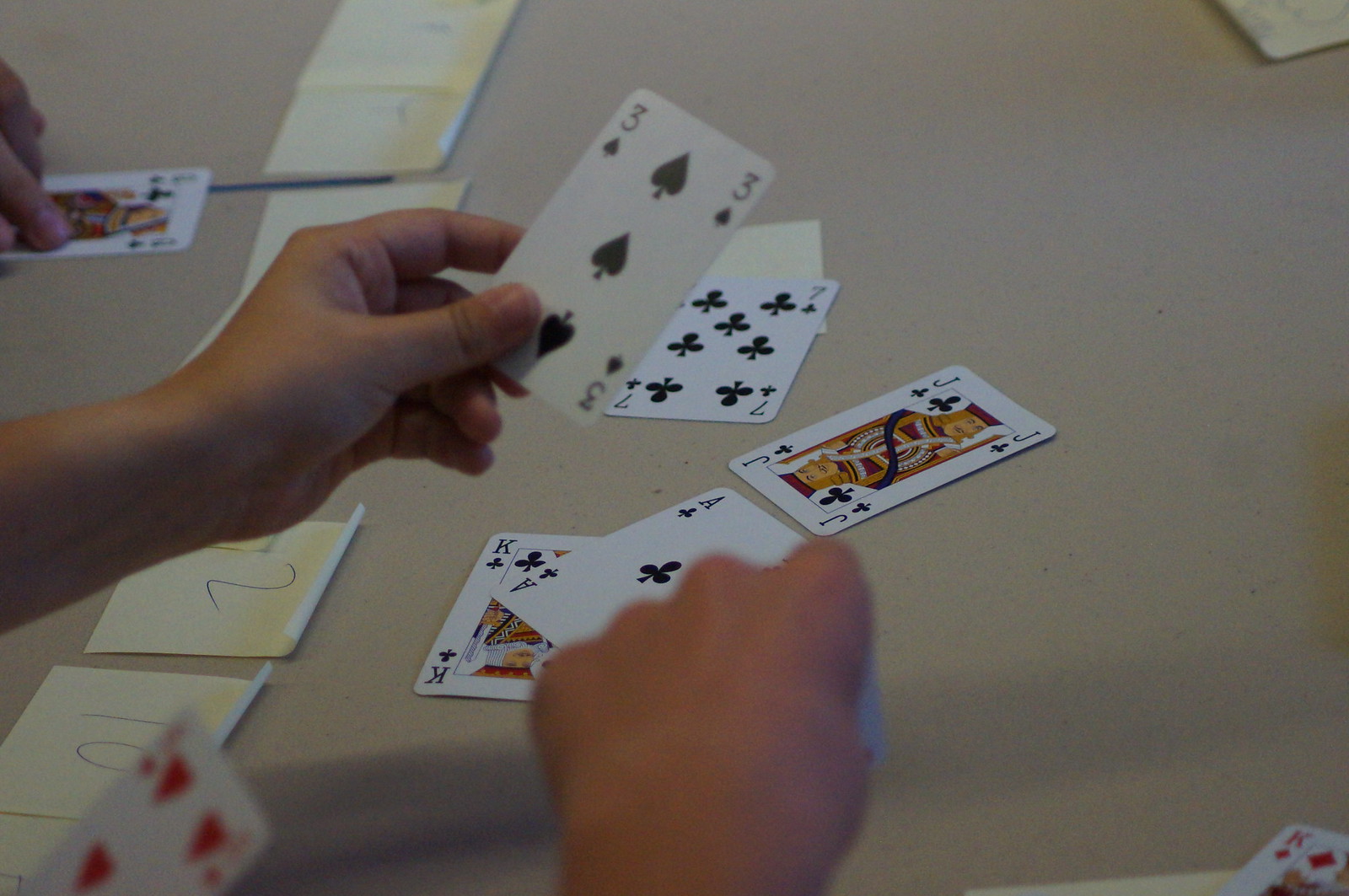In this image, a white or off-white table or counter, possibly with light speckling, serves as the setting for a card game. Multiple hands are visible, suggesting the presence of at least three players. One person's hands are prominently positioned in the bottom middle of the frame, while another player's hand emerges from the left side, and a third individual's fingers appear at the top left corner. 

Each player has a spread of playing cards before them. One player is holding a black 3 of spades, while visible cards also include the jack of clubs, ace of clubs, king of clubs, and seven of clubs, along with an indistinct hearts card. Additionally, white square pieces of paper or sticky notes, some bearing numbers such as 10 and 2 (with an unclear preceding digit), are scattered on the table. The players' focused postures and the organized array of cards and numbered notes suggest they are engrossed in a strategic card game, though the specific game remains unidentified.